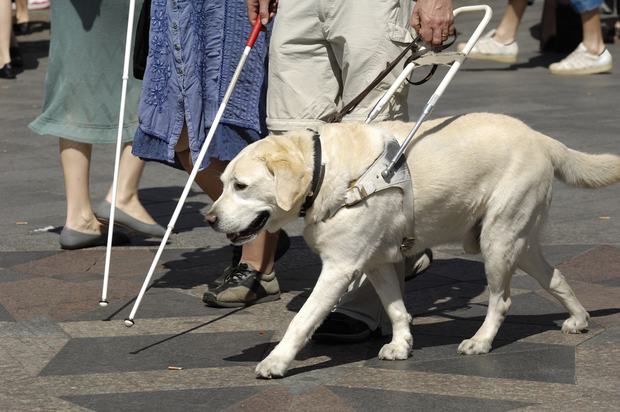In the photograph, a light yellow Labrador Retriever, equipped with a white leather harness and a sturdy metal handle, guides a man who is holding both the harness and a thin white cane, indicating his visual impairment. The man is wearing white shorts, and the image only shows up to his waist. To his left, two additional people are visible in part: a woman in a blue dress, also holding a white cane, and another pair of ankles and shoes walking leftward in the upper right corner. The scene takes place on a cemented street, dotted with a few cigarette butts, and the dog appears focused and in mid-stride, diligently performing its duties as a guide dog.